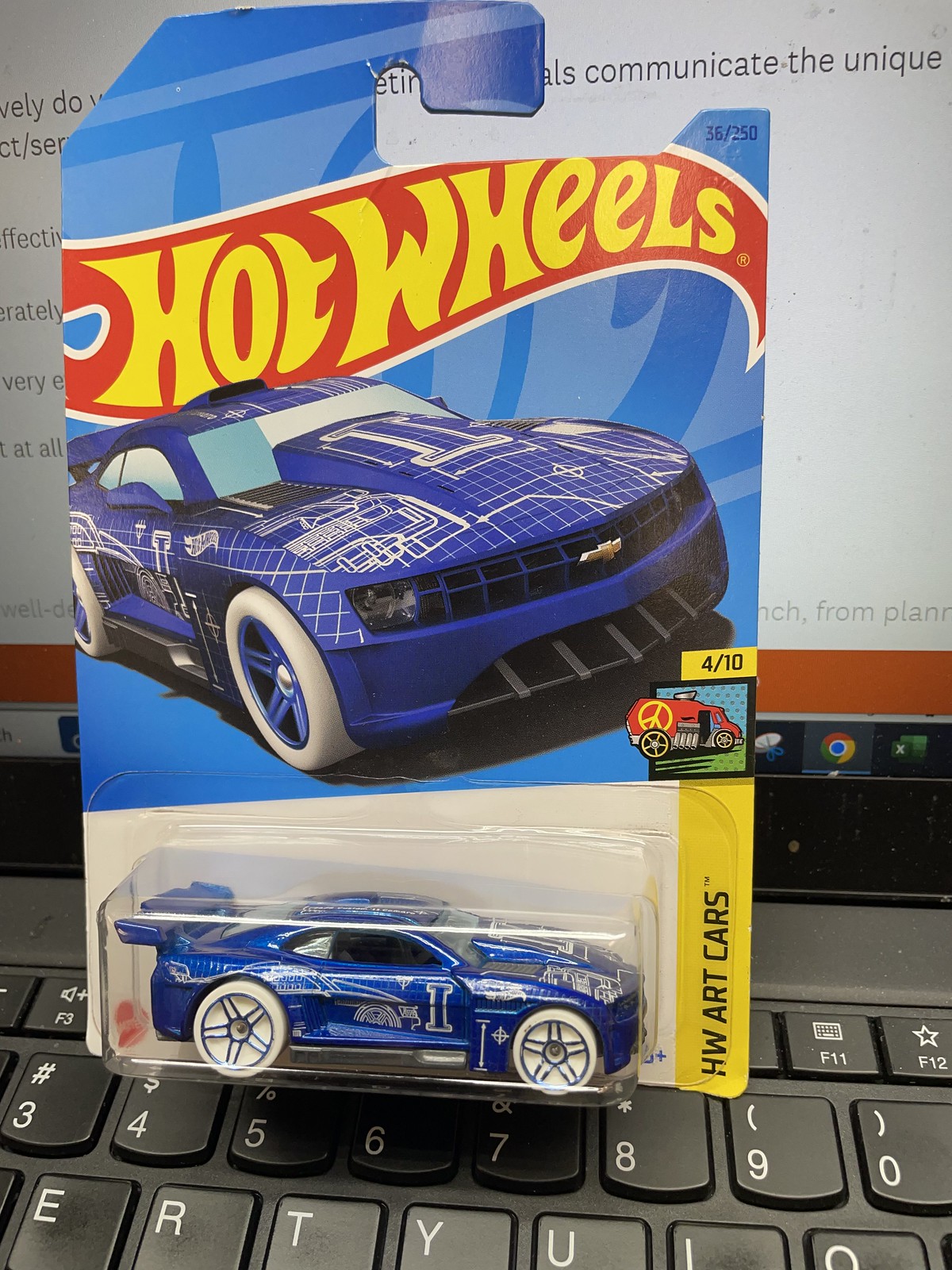This rectangular photograph captures a close-up view of a Hot Wheels toy car package placed on top of a laptop keyboard, with its top part leaning against the laptop screen. The computer screen acts as a white background for the upper half of the image, displaying some text, while the lower half features the black keyboard.

The focal point of the image is the Hot Wheels package, which prominently displays a blue sports car adorned with a futuristic, technology circuit grid blueprint-like paint design and white wheels. The toy remains encased in its clear plastic cover, attached to a cardboard backing. Above the plastic encasement, the Hot Wheels logo, characterized by a red banner with yellow lettering, is clearly visible.

The package art includes a detailed illustration of the blue sports car driving towards the viewer from the left to the lower right. On the right-hand side, the text "HW Art Cars" is printed in black on a yellow strip. Additionally, the packaging indicates that this specific car is "4 out of 10." Beneath this, there is also a small illustration of a red van-like vehicle with a hot rod engine, although the actual toy car in the package matches the blue sports car design.